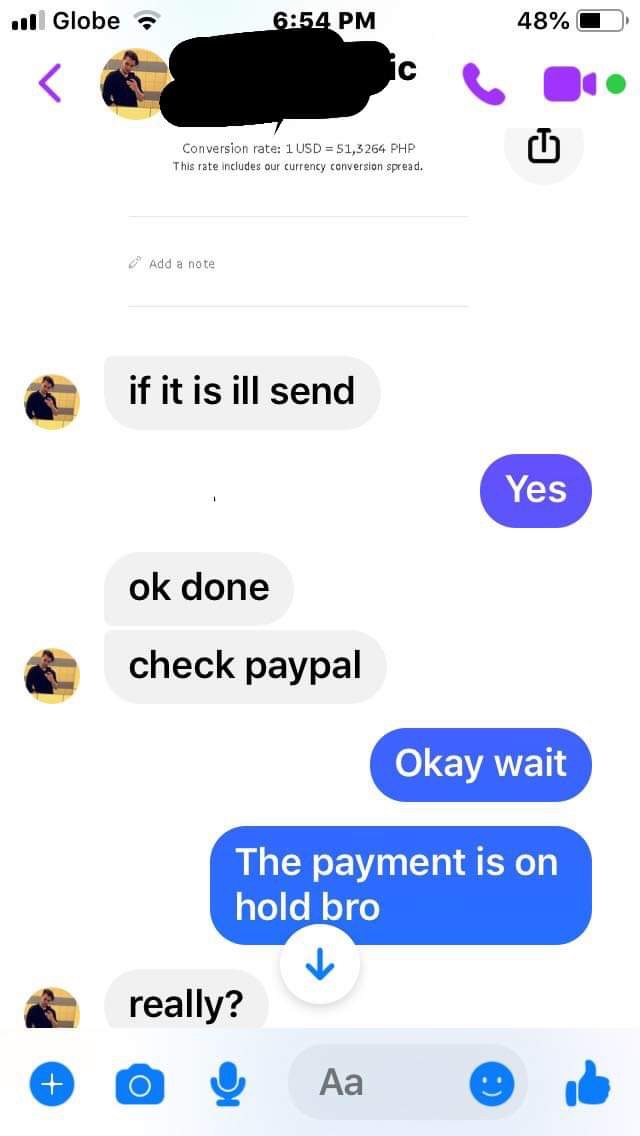The image displays a screenshot of a Facebook Messenger conversation on an iPhone, held at 6:54 PM with 48% battery life. At the top left of the screen, it shows three reception bars, the word "Globe," and Wi-Fi connectivity. A profile picture and name have been obscured by the user who took the screenshot. Below, the conversation unfolds in black text with a gray background for one participant and white text on blue bubbles for the other. The exchange starts with, "If it is, I'll send," followed by the response, "Yes." The initial sender then says, "Okay, done. Check PayPal," to which the recipient replies, "Okay, wait." The conversation continues with, "The payment is on hold, bro," and ends with the sender's exasperated "Really?" At the bottom of the screen, traditional messaging icons are present, including the attachment, photo, voice recording, emoji, thumbs up buttons, and a text input field. A small, unidentifiable black object appears at the top of the image, possibly related to a USB device.